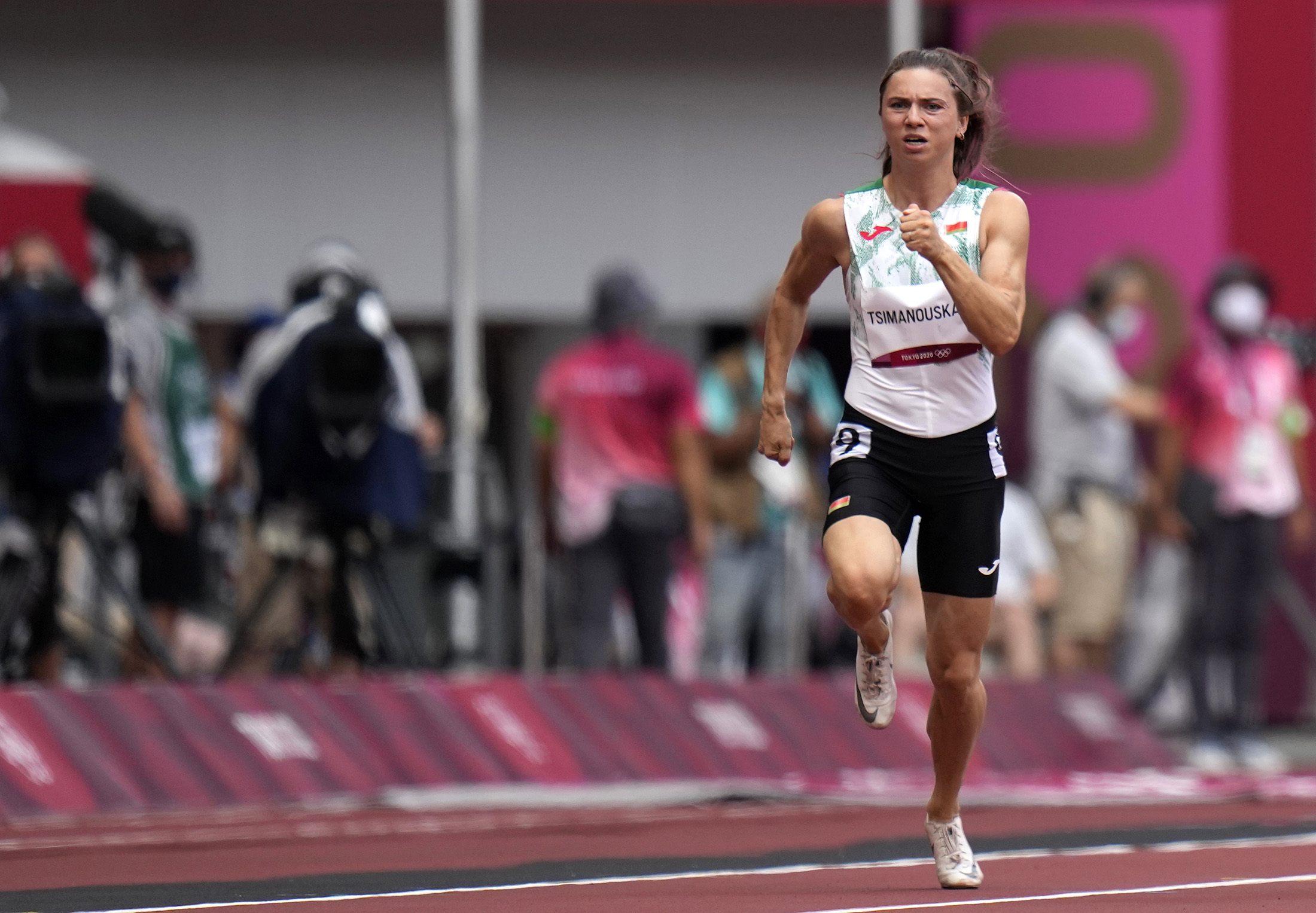The image features a highly focused shot of a female athlete competing in a race on a red clay track marked with white lines. The background, blurred, shows figures that are likely spectators or officials, making the athlete the central figure. She is positioned on the right side of the image, running with determined focus. She is a white woman with brown hair tied in a ponytail, and she is wearing a white tank top with a green and white racing bib emblazoned with "Tsimanouskaya" in black letters. She also sports black shorts, black shorts displaying the number 9, and white Nike shoes. The athlete wears an earring, accentuating her athletic yet determined appearance. The detailed elements of the attire and track capture the intensity and atmosphere of the racing event.